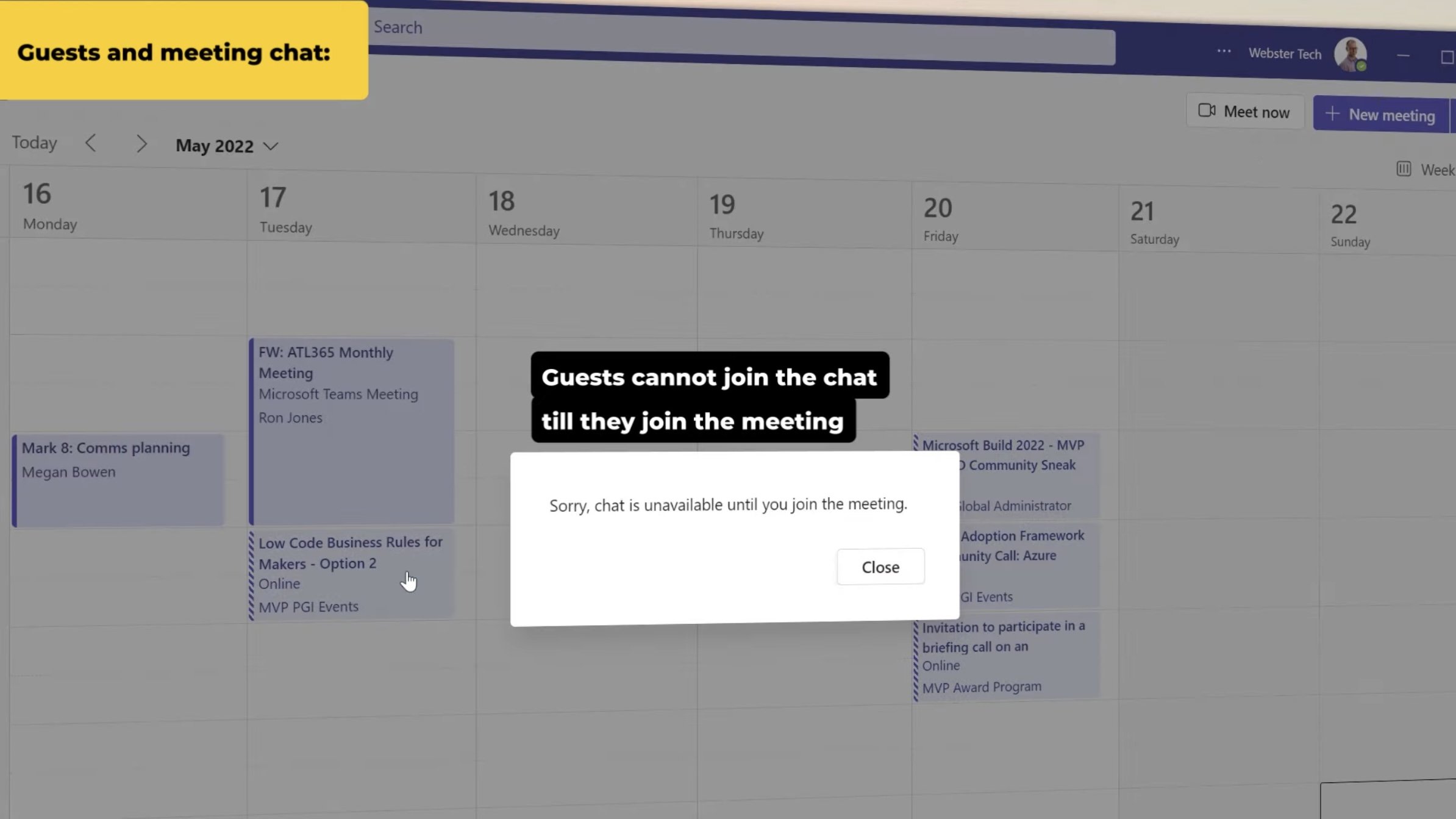A detailed caption for the image:

The image depicts a screenshot of a chat website. The interface is divided into two main sections. In the background, there is a calendar primarily colored in blue and white, displaying a weekly view from Monday the 16th to Sunday the 22nd. At the top of the calendar is a search box. The calendar includes various scheduled items, such as a meeting on Monday the 16th titled "Mark 8th meets Megan Bowen," suggesting it's a work-related calendar.

Superimposed on this calendar is a prominent white box, indicating an ongoing user interaction. This active box contains the message, "Sorry, chat is unavailable until you join the meeting," along with a "Close" button at the bottom. Above this active box, there's a black text box with white text that reads, "Guests cannot join the chat until they join the meeting," providing context for the chat's inaccessibility. Additionally, there's another notification box labeled "Guest and meeting chat," reinforcing the requirement to join the meeting to participate in the chat. The overall scenario suggests that the user attempted to access a chat feature tied to a scheduled meeting but encountered restrictions due to not having joined the meeting yet.